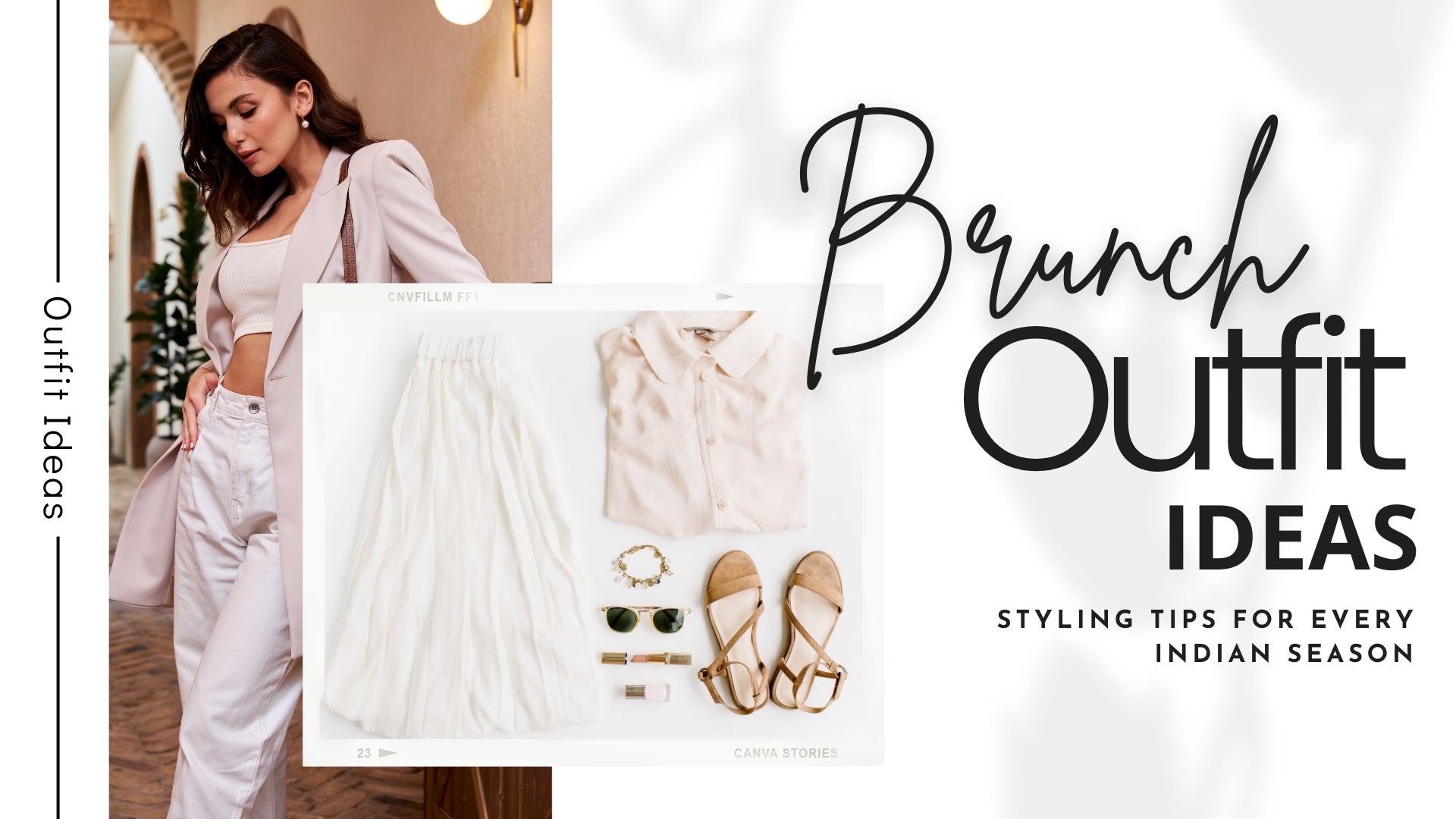This is an online digital advertisement for brunch outfit ideas and styling tips for every Indian season. Featured on the left side is an image of an elegant Indian woman with long brown hair, wearing a cream-colored crop top, high-waisted white pants, and a small cream-colored blazer. She stands inside a building with an archway and cream-colored walls, her right hand casually slipped into her pocket. A pearl earring dangles from her left ear as she looks slightly down, facing slightly to the right. Superimposed above her is an assortment of outfit items laid out, including a white skirt, a cream-colored blouse, brown sandals, sunglasses, a bracelet, and possibly a belt, all exuding the same chic and minimalist vibe. A thin vertical stripe of black runs along the left edge of the image, with the words "Outfit Ideas" outlined in black and placed sideways within it. On the right side of the advert, in cursive script, are the words "Brunch Outfit Ideas," followed by "Styling tips for every Indian season" in black print.